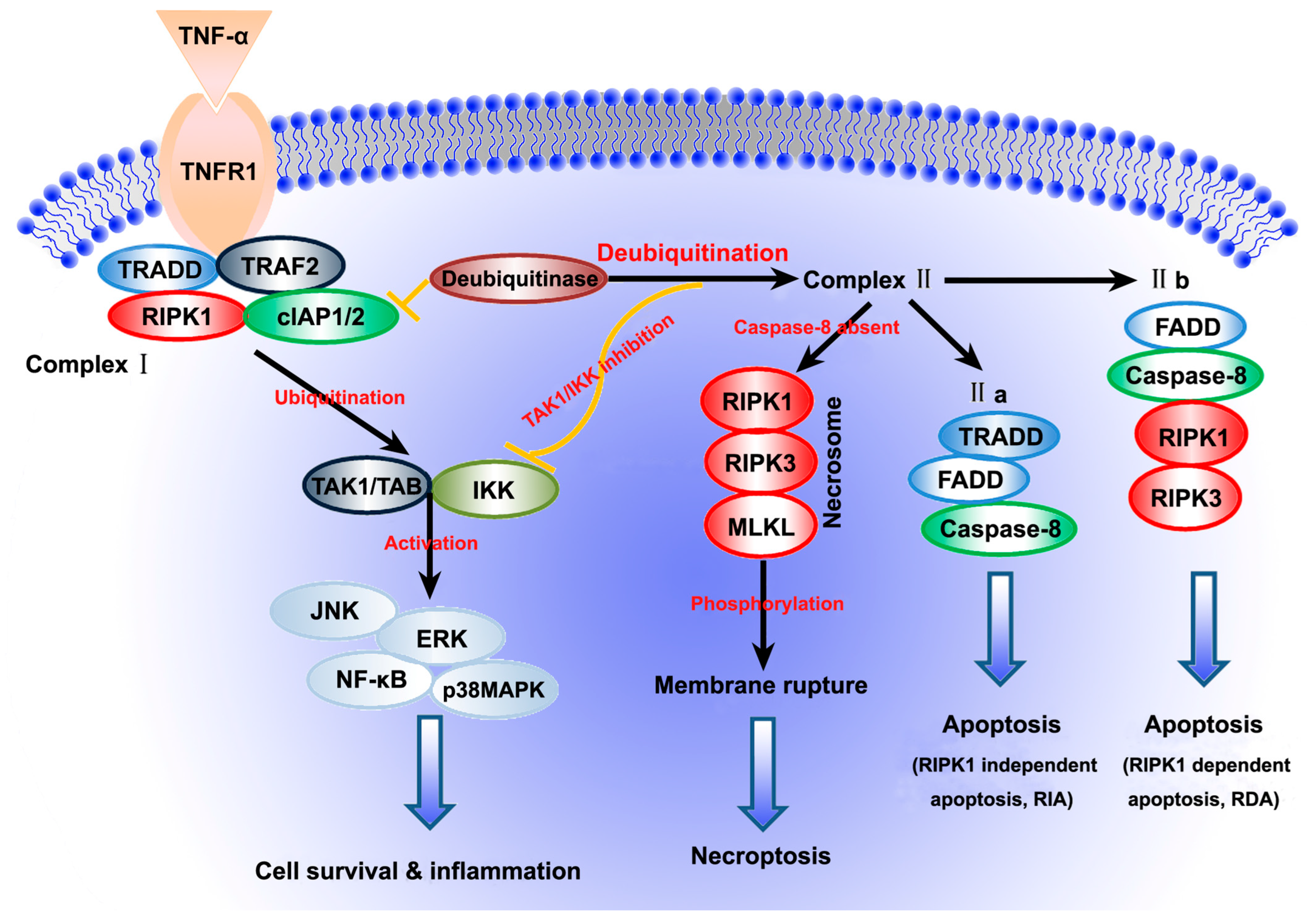This horizontal image presents a detailed, multicolored flow diagram set against a bluish-purple background at its center. Dominating the top of the image is a dotted blue banner with two rows that feature thin lines converging but not quite meeting. In the upper left, an inverted brown triangle labeled "TNF-alpha" leads into an oval marked "TNF-R1."

Below this, four ovals labeled "TRADD," "TRAF2," "RIPK1," and "Complex 1" are prominently featured, with black text inside and arrows connecting them. These structures converge and channel information downwards, culminating in elements that indicate "cell survival" and "inflammation."

Further down the diagram, another element labeled "Complex 2" is prominently highlighted, with three distinct pathways branching out from it. These pathways represent "necroptosis," "apoptosis," and "apoptosis with independent and dependent RIA and RDA," respectively, detailing different cellular outcomes. The lower portion of the image features four distinct products, summing up the diagram's processes and flows.